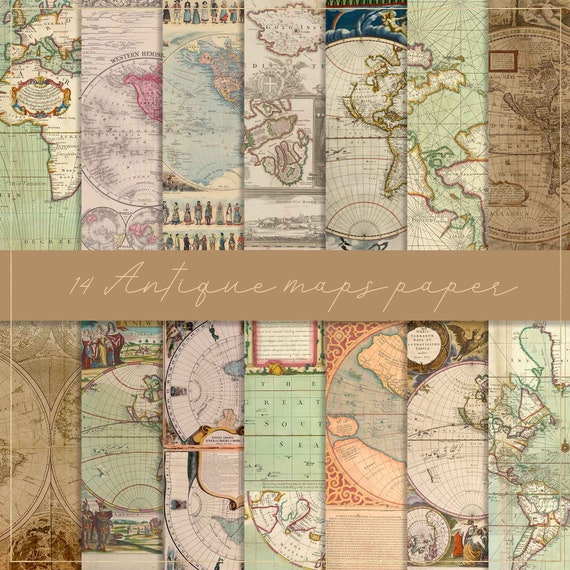The image depicts a cover of a book titled "14 Antique Maps Papers." The central text, written in cursive in a beige hue, is set against a light brown rectangle. Surrounding this text is a diverse array of map illustrations, each rendered in unique colors and styles. These maps showcase different parts of the world, such as Africa, Asia, Europe, North America, and South America. Some maps feature half-globes with colored blue oceans and distinct continents, while others have more historical, vintage looks, including black and white line drawings and oxidized brown hues. The variety of illustrations spans from top to bottom, creating a rich collage that highlights various cartographic depictions and worldviews. In the top left corner, notably, are depictions of Africa and Asia. The number "14" is prominently displayed next to the word "Antique" on the left side.